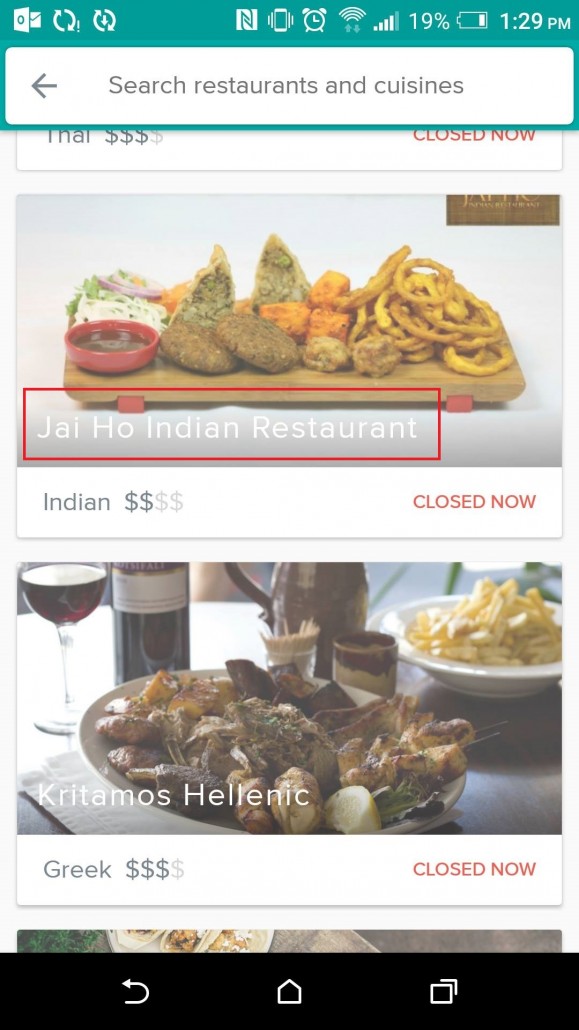This appears to be a screenshot from a mobile device. At the top of the screen, there is a green status bar displaying various mobile icons in white, including Wi-Fi signal strength, battery at 19%, and the current time, 1:29 PM. Directly below this is a white rectangular search bar highlighted with a green border, featuring a grey arrow on the left and the placeholder text "Search Restaurants and Cuisines."

Below the search bar are two photographs. The first image showcases a spread of Indian food arranged on a wooden board. Overlaying this image are the words "Jai Ho Indian Restaurant," written in white font on a grey background, and the text is further accentuated by a red rectangular border. Beneath this, it is indicated that the restaurant specializes in Indian cuisine and currently has a status of "closed now," displayed in red font.